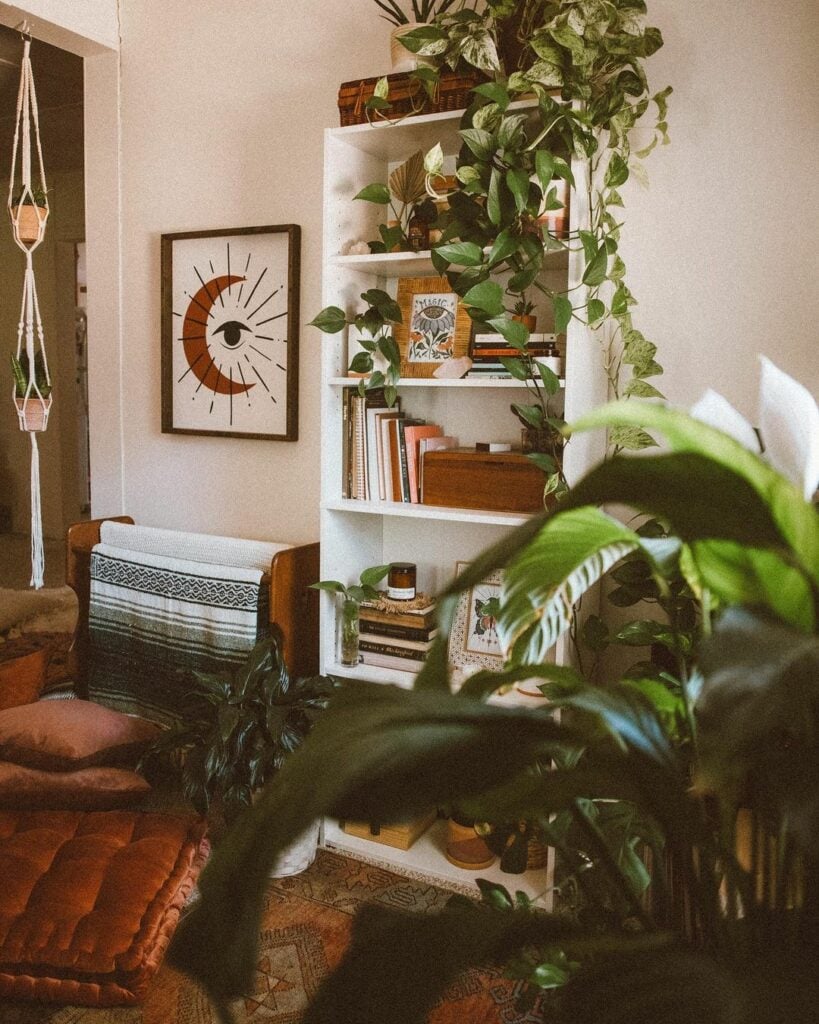The image depicts a cozy living room with white walls, dominated by a centrally placed white bookcase. This six-tiered bookcase is adorned with a lush, trailing vine plant at the top, which drapes elegantly down the shelves, adding a touch of vibrant greenery. The top shelf also houses a decorative basket. The subsequent shelves are filled with various items: the second shelf, partially obscured by the vines, contains a couple of crystals; the third shelf features a framed picture of flowers and a small potted plant sitting on a stack of books; the fourth shelf has books and notebooks stacked horizontally alongside a small chest that holds another potted plant; the fifth shelf has another stack of books with a glass jar on top, a potted plant in front, and a framed picture (possibly of a butterfly); and the bottom shelf contains what looks like an opening box and a couple of baskets, mostly hidden by a foreground plant.

To the right of the bookcase stands a brown blanket holder draped with a white and striped blanket. Above the blanket holder hangs a framed artwork of a crescent moon with an open eye at its center, emanating star-like lines. This piece of art adds an eclectic touch to the room.

The floor is covered with a rich brown tapestry rug, accompanied by several plush brown pillows. The space is further enhanced by hanging plants and decorative baskets on the walls, contributing to the room's abundant greenery. In the foreground, a tall plant partially obscures the view of the bookcase, reinforcing the room's lush, verdant atmosphere. The overall scene is a harmonious blend of cozy furnishings and natural elements, creating a serene and inviting living space.